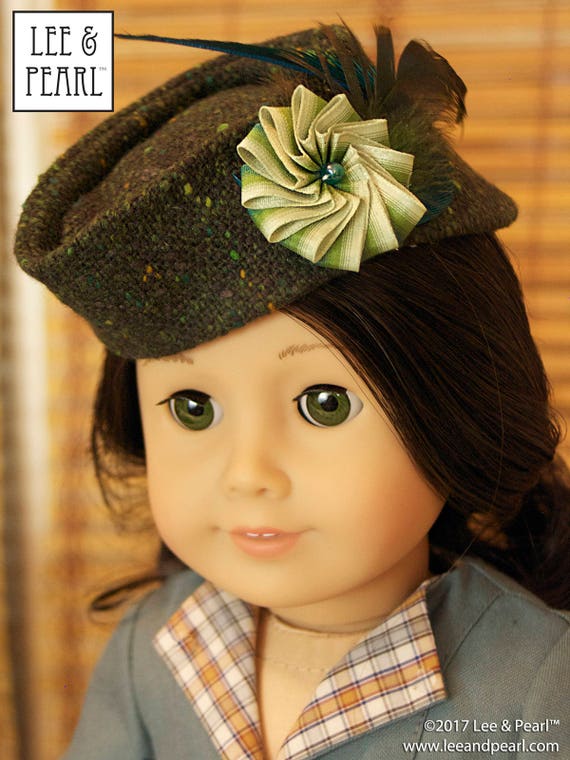In this color photograph, a collectible doll resembling an American Girl doll is centered in front of light brown mini blinds. Facing slightly to the left, the doll has long brunette hair pulled back from her face and striking green eyes. Her lips smile softly, showing her two front teeth in a peach hue. She wears a brown hat adorned with a green rosette on the side and a feather that curls toward the front. Her outfit includes a gray jacket with pin tucks on the shoulders and a collared shirt featuring a vibrant plaid pattern of green, orange, and white.

In the top left corner of the image, a white box with a black border prominently displays the text "LEE & PEARL" in capital letters, with a trademark symbol next to "LEE." The bottom right corner bears a copyright notice that reads, "© 2017, Lee & Pearl™ www.leeandpearl.com," all in white lettering. The overall style of the doll suggests a vintage, 1920s-inspired appearance.